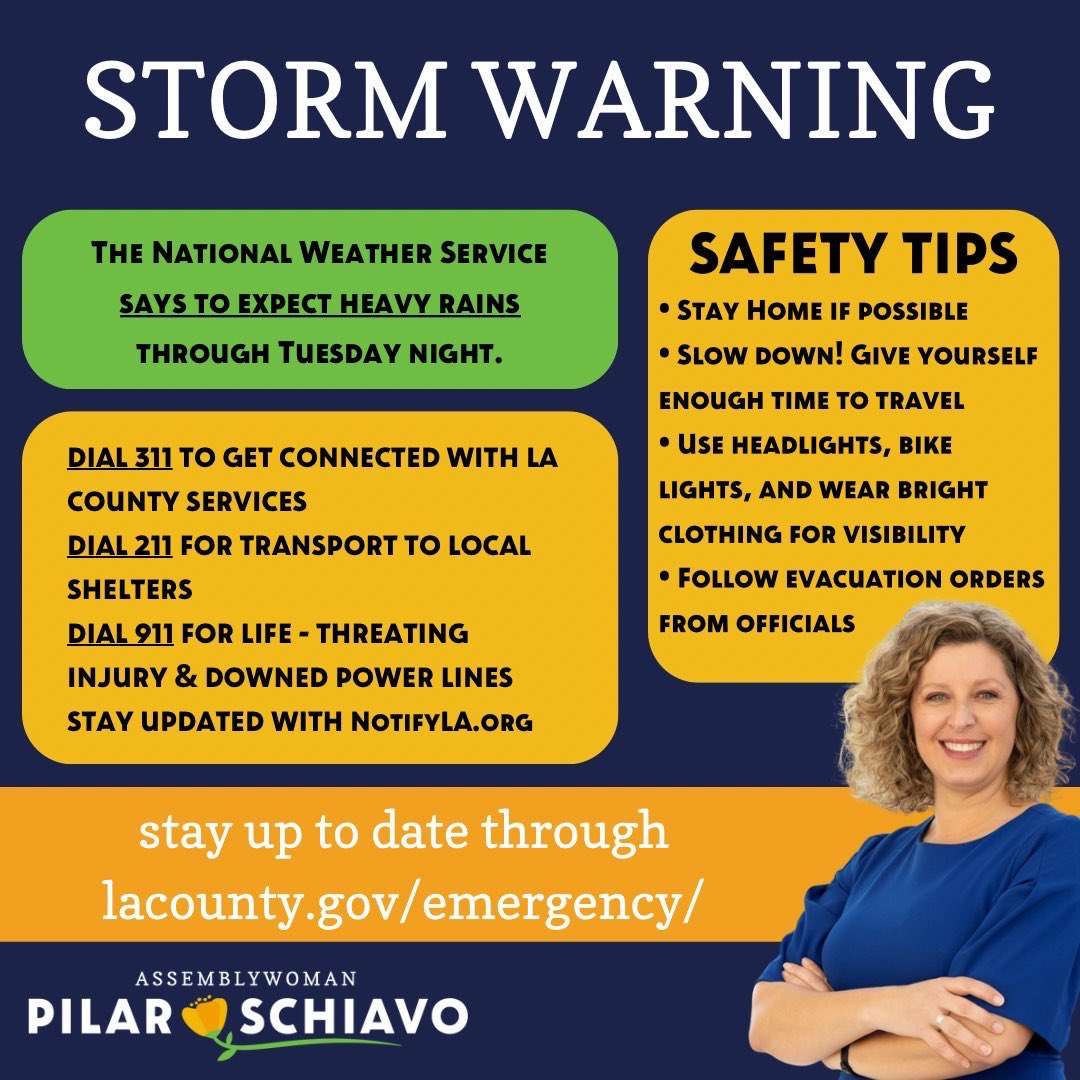The image is a public service announcement flyer featuring a storm warning. The top of the flyer prominently displays "Storm Warning" in bold white text on a black background. Below, a green box states, "The National Weather Service says to expect heavy rains through Tuesday night." Adjacent to it, a yellow box provides essential contact information: "Dial 311 to connect with LA County Services, dial 211 for transport to local shelters, dial 911 for life-threatening injuries and downed power lines. Stay updated with notifyLA.org." 

To the right, a vertical orange box outlines safety tips: "Stay home if possible, slow down, give yourself enough travel time, use headlights and bike lights, wear bright clothing for visibility, follow evacuation orders from officials." A horizontal golden bar underneath reads, "Stay up to date through lacounty.gov/emergency."

At the bottom left corner, the flyer features the name "Assemblywoman Pilar Schiavo" separated by a yellow flower. On the right, a photograph captures Pilar Schiavo, a smiling woman with short blonde curly hair, wearing a blue shirt and crossing her arms. The flyer emphasizes staying informed and safe during the upcoming storm.